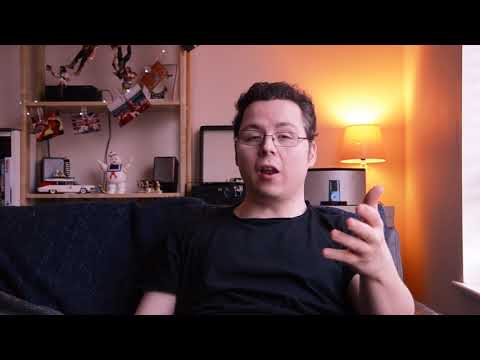In the photo, a man wearing black-framed glasses and a black t-shirt is seated on a dark blue or black couch, facing the viewer. His left hand is raised and fingers splayed, while his mouth is open, suggesting he is speaking. Behind him, over his left shoulder, a lit lamp projects light onto the wall, illuminating a wooden shelf. The shelf holds several collectible figurines, notably including the Stay Puft Marshmallow Man and the Ghostbusters' Ecto-1 car. The background also features a series of photos hanging near the shelf, and a possible mini-fridge is visible next to the lamp. The walls are a tan or cream color, and there is a black line across the top and bottom of the image. This setting appears to be a personal space, likely a room where he displays his collection and spends time.